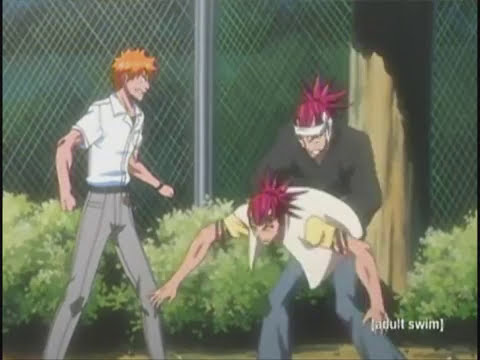This image is a highly detailed screenshot from an animated television show, possibly a cartoon featured on Adult Swim. It portrays a dramatic scene involving three white male characters, seemingly in the midst of a conflict. The setting is delineated by a tall, dark gray or silver chain-link fence in the background, with green shrubs and grass visible both behind and in front of the fence. The right side of the image showcases a brown tree trunk.

In the foreground, the leftmost character stands assertively with legs apart, dressed in a white short-sleeve button-down shirt and gray pants. He has short orange hair and appears to be angered, seemingly directing his hostility toward the other two men.

The central character is hunched over, indicating he might be in distress or off-balance, wearing a white shirt and gray pants, with his arms outstretched as if trying to prevent a fall.

The third man, positioned behind the hunched figure, seems to be shoving him. This character is attired in all black, featuring spiky bright red hair, contributing to the intense and animated atmosphere of the scene.

Overall, the intricate background and vivid character descriptions suggest a moment of intense action, characteristic of animated television programs. The presence of the "Adult Swim" logo in the bottom right corner confirms its likely source.